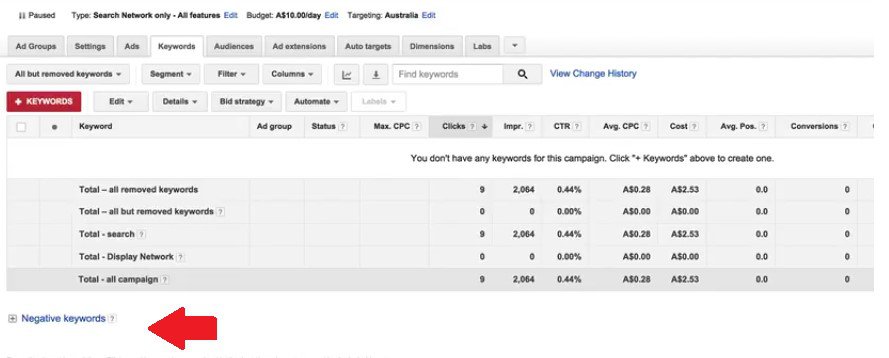Here we have a screenshot from a webpage that displays an email-like interface. At the top, there are two bold black lines; the first line states "Paused" and the second says "Type". Following this, in bold black text, we see "Search Network Only - Features" with a hyperlinked blue "Edit". Below, it reads "Budget" in black, followed by "$10.00/day", where "$" likely denotes Australian Dollars due to subsequent contextual indicators. The "Budget" section also has a blue "Edit" hyperlink. Further down, another section marked "Targeting" in blue states "Australia", confirming the dollar signs indicate Australian dollars. This section too has an "Edit" hyperlink.

Directly below is a navigation tab bar. The unselected tabs, which have a mid-grey background and black text, are labeled: Ad Groups, Settings, Ads, and Audiences. The currently selected tab, "Keywords", is highlighted in white. Additional unselected grey tabs include Ad Extensions, Auto Targets, Dimensions, and Labs.

Separated by a thin grey line, there is a dropdown element labeled "All but Removed Keywords" in bold black with a black drop-down arrow. Nearby, there are other dropdown elements named Segment, Filter, and Columns. Icons following these dropdowns include a square with an "L" squiggle and another square with an arrow.

On the right side, there's a rectangle with a bold black border containing a light grey square with a dark black magnifying glass. A search bar in the center reads "Find Keywords" in grey text. Adjacent to it, on the left side, is a red rectangular button with bold white text and a plus symbol that reads "Keywords".

Below, there are multiple mid-grey rectangular buttons labeled Edit, Details, Bid Strategy, Automate, and Labels in dark grey text. The Labels button features a dropdown arrow.

Further into the interface, there is a section organized like an email setup but appears to be in 'Settings'. Here, various elements are partitioned by thin grey lines. Each section title is in bold black text. The first section titled "Ad Groups" includes sub-sections such as "Ad Group Status" with dropdowns featuring grey question marks. Other columns within this section display data metrics such as "Max. CPC", "Clicks", "CTR", "Average. CPC", "Cost", "Avg. Pos.", often with accompanying tooltips denoted by question marks.

The interface contains grey rectangles with black text saying "Total - All Removed Keywords" on the left and corresponding numerical metrics such as 9, 2064, 0.44%, 0.28 AUD, and 2.53 AUD on the right. Similarly, it displays "Total - All but Removed Keywords" and "Total - Search" with corresponding data columns, each followed by a "?" icon offering explanations.

The "Total Display Network" section shows zeros across all columns. Finally, "Total - All Campaigns" is highlighted with a darker grey bezel and provides summarized campaign statistics, emphasizing figures like 0.28 and 2.53 AUD.

At the bottom right, the display features a red arrow pointing to hypertext in blue labeled "Negative Keywords", next to a grey square with a plus symbol and a dark grey interior question mark.